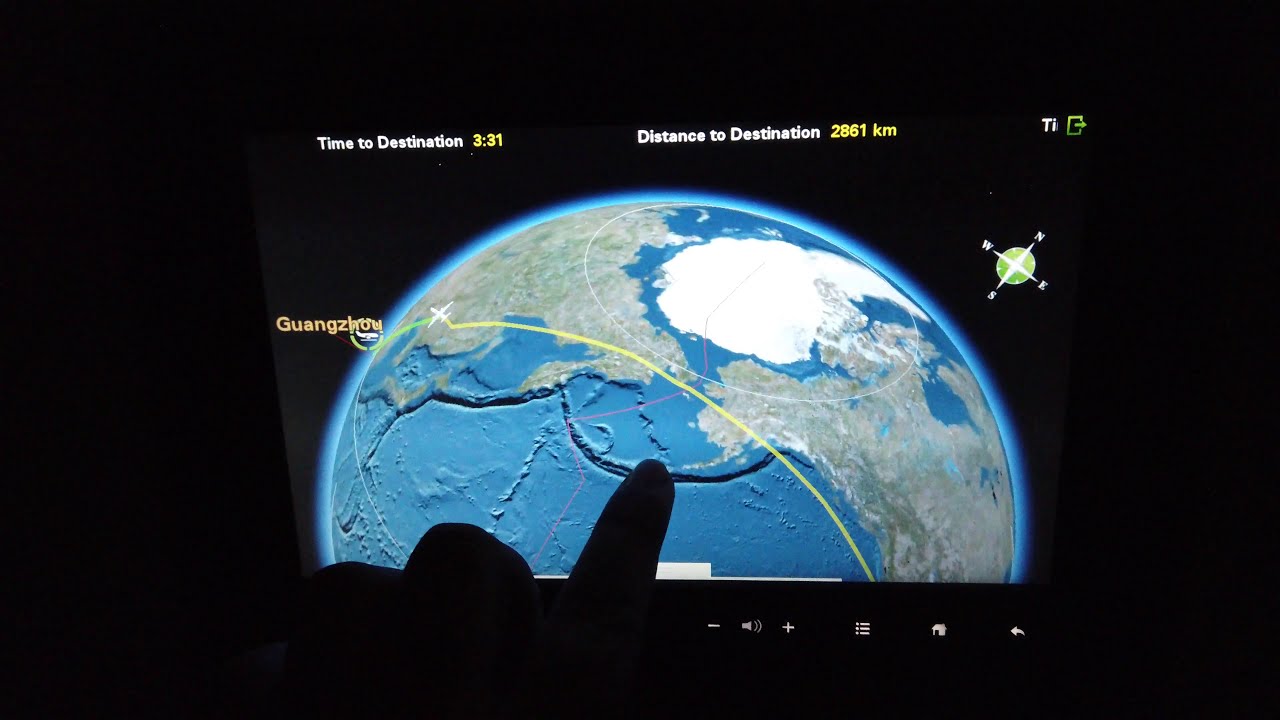The photograph captures a dimly lit in-flight plane tracker screen, surrounded by darkness, with the silhouette of a person’s hand prominently displayed on the left, their forefinger extended and pointing at the screen. The illuminated screen shows a 3D view of the Earth, prominently depicting the curvature of the northern hemisphere with blue oceans and brown landmasses, along with white representing ice at the North Pole. A yellow flight path arcs across the globe from North America over Alaska and Russia toward Guangzhou, China, indicated by "Guangzhou" in orange text on the left side of the screen. The tracker also displays a white plane icon mid-route. On the right side, a green compass with white directional points is visible, oriented with north pointing to the top right corner. Top screen text reads "Time to destination: 3:31" and "Distance to destination: 2,861 kilometers." Additional information such as a door icon with "Ti" appears in the top right. At the bottom, the screen features multiple control icons including volume, menu, home, and back.